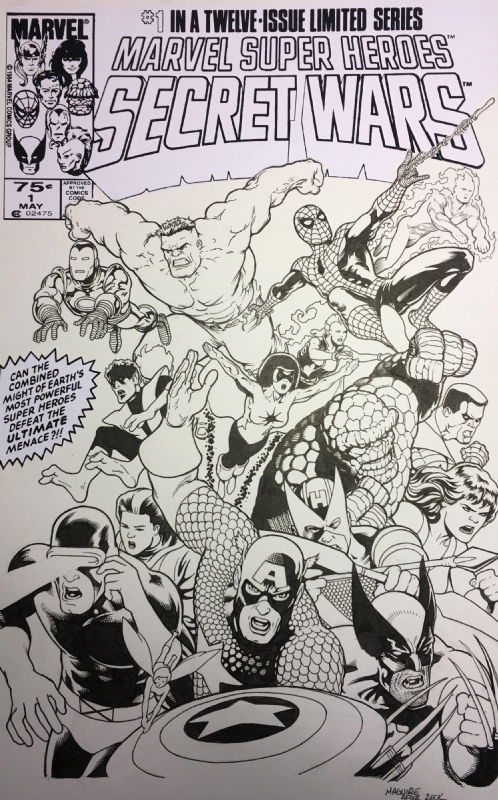This image showcases the front cover of the comic book "Marvel Super Heroes Secret Wars," number one in a 12-issue limited series. The cover is entirely black and white and prominently features an array of Marvel characters, including Spider-Man, Captain America (indicated by the "A" on his head), Iron Man, and the Hulk, amidst a backdrop of dynamic action. The central theme of the cover reveals superheroes engaged in various activities such as flying, running, and Spider-Man shooting webs. 

The text on the cover reads "Marvel Super Heroes Secret Wars" in bold white letters outlined in black, and further specifies it as number one in the series. The price is marked as 75 cents, and it is dated May 1st. Additional text on the cover poses a gripping question: "Can the combined might of Earth's most powerful superheroes defeat the ultimate menace?" This text is set against a jagged backdrop, enhancing the drama of the declaration. Various tools and weapons are in the characters' hands, adding to the sense of imminent battle and high stakes.